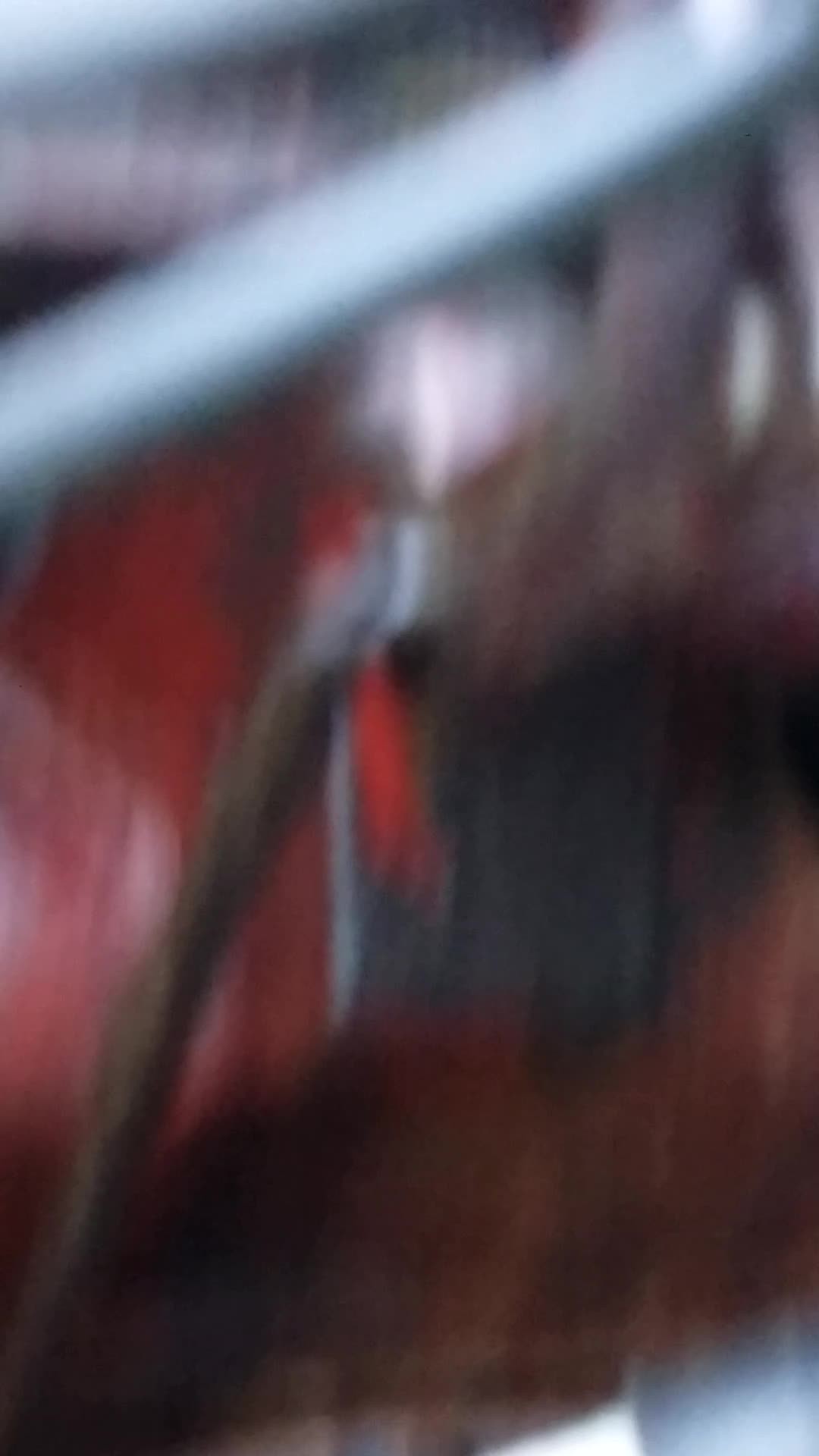This image, presented in narrow portrait mode, is an abstract blend of blurred colors. Dominating the scene is a diagonal swath of light blue, beginning about a third of the way down from the left edge and extending towards the upper right corner. Below this blue band, there are significant smudges of red, adding a striking contrast. A slender, brown shape also cuts across the composition, originating from the lower left corner and diagonally progressing towards the center right before tapering off. The background colors vary, featuring shades of gray and dark gray, with patches of white interspersed throughout. The image is highly unfocused, rendering the subjects unidentifiable and contributing to its abstract, dream-like quality.